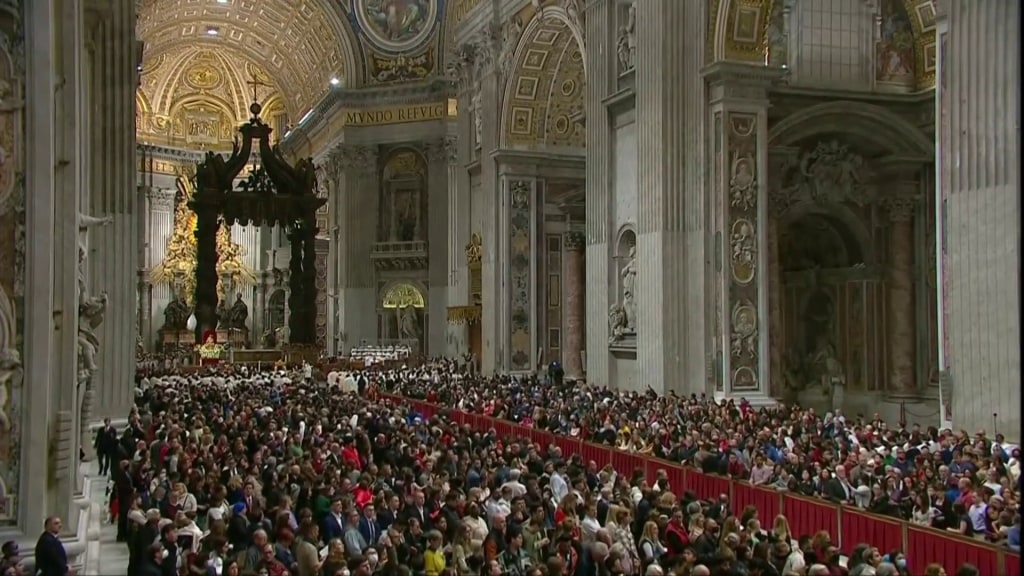The image depicts a grand, highly ornate interior of a large cathedral, possibly a famed structure like Westminster Abbey or St. Peter's Basilica. The setting is adorned with high ceilings, gold emblems, and intricate arches and pillars, contributing to its majestic atmosphere. Positioned at the end of the hall is a figure, potentially the Archbishop of Canterbury or the Pope, seated on an opulent red velvet throne. The cathedral is filled to capacity with an immense crowd of people, numbering in the hundreds, all packed tightly into the pews. A red barrier, likely gates, runs down the center aisle, further dividing the crowd into two sections. The massive gathering is viewed slightly from above and at an angle, showcasing a sea of people in various colored outfits. On the left side, beyond the red barrier, there is a stout concrete wall that transitions from white at the bottom to a darker brown at the top, featuring an archway. The decorative elements continue with golden accents and intricate markings adorning various parts of the walls and ceiling, adding to the overall grandeur of the scene.